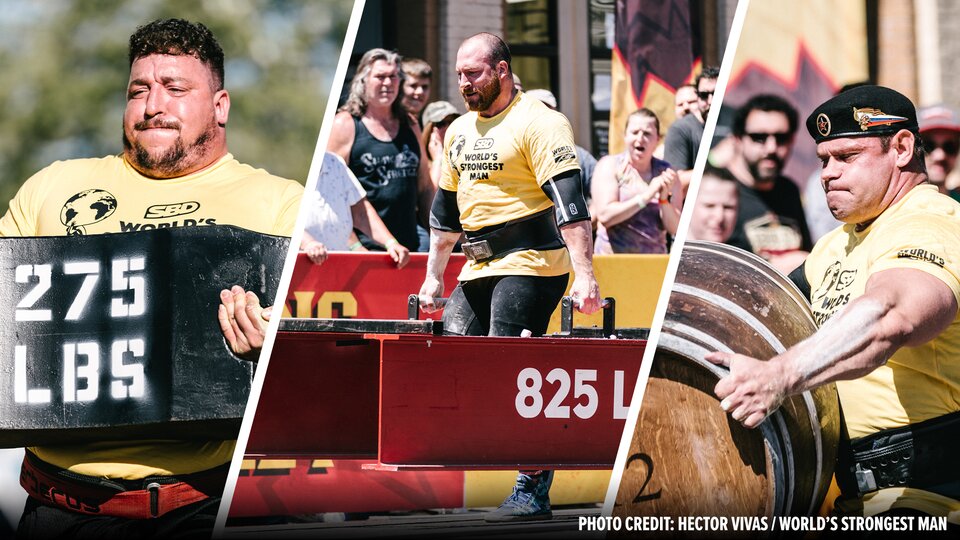This is a photo collage from the World's Strongest Man competition, featuring three distinct frames of athletes demonstrating immense strength. Each competitor is wearing a yellow jersey with the "SBD" logo and an image of the Earth being lifted by a hand, symbolizing their incredible feats of strength. On the left, a man with a strained expression is lifting a large black box labeled "275 pounds." The middle frame showcases another powerlifter, equipped with a weightlifting belt, gripping handles of a hefty 825-pound weight. Finally, the rightmost image depicts a strongman hoisting a substantial barrel, his face contorted with the sheer effort. A cheering crowd in the background emphasizes the event's excitement and high energy. Photo credit: Hector Vivas.